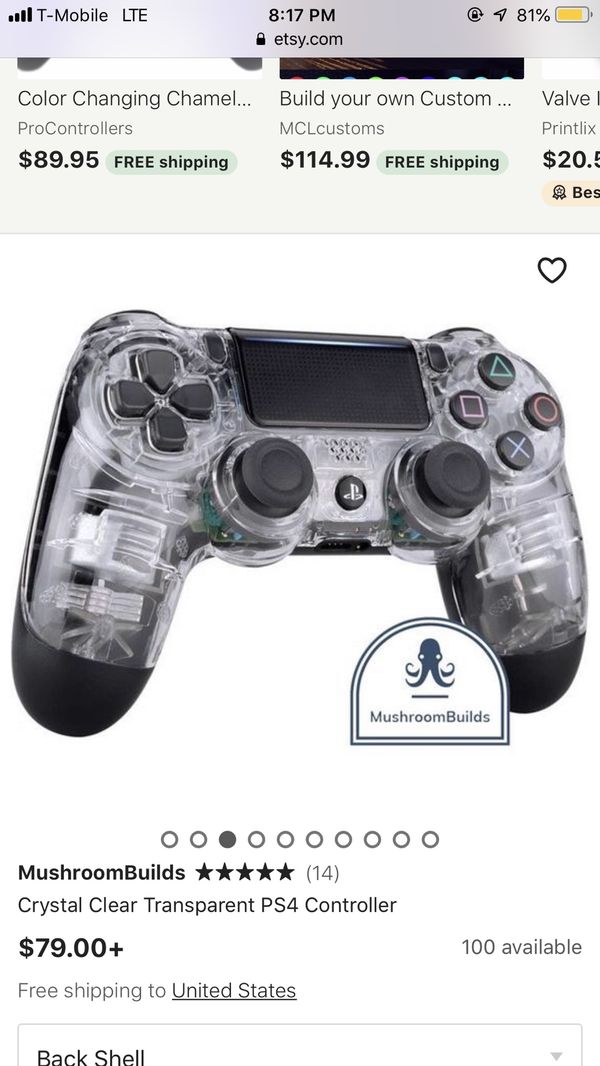This is a screenshot taken from a mobile device, displaying a shopping webpage on Etsy. The screenshot does not include the physical device, only the screen's content. At the top of the screen, standard mobile device icons are visible, including network connection, time, and battery status, along with a black padlock icon and the web address etsy.com. The webpage appears to be a product listing with the top section partially cut off due to scrolling.

The main content of the image shows a thumbnail grid of various products with their names, prices, and shipping costs. Dominating the lower part of the screenshot is a large image of a PlayStation controller with a see-through case, revealing its inner components. This product image features a watermark for a company named Mushroom Builds, accompanied by an octopus logo. The listed product is described as a "Crystal Clear Transparent PS4 Controller" priced at $79.